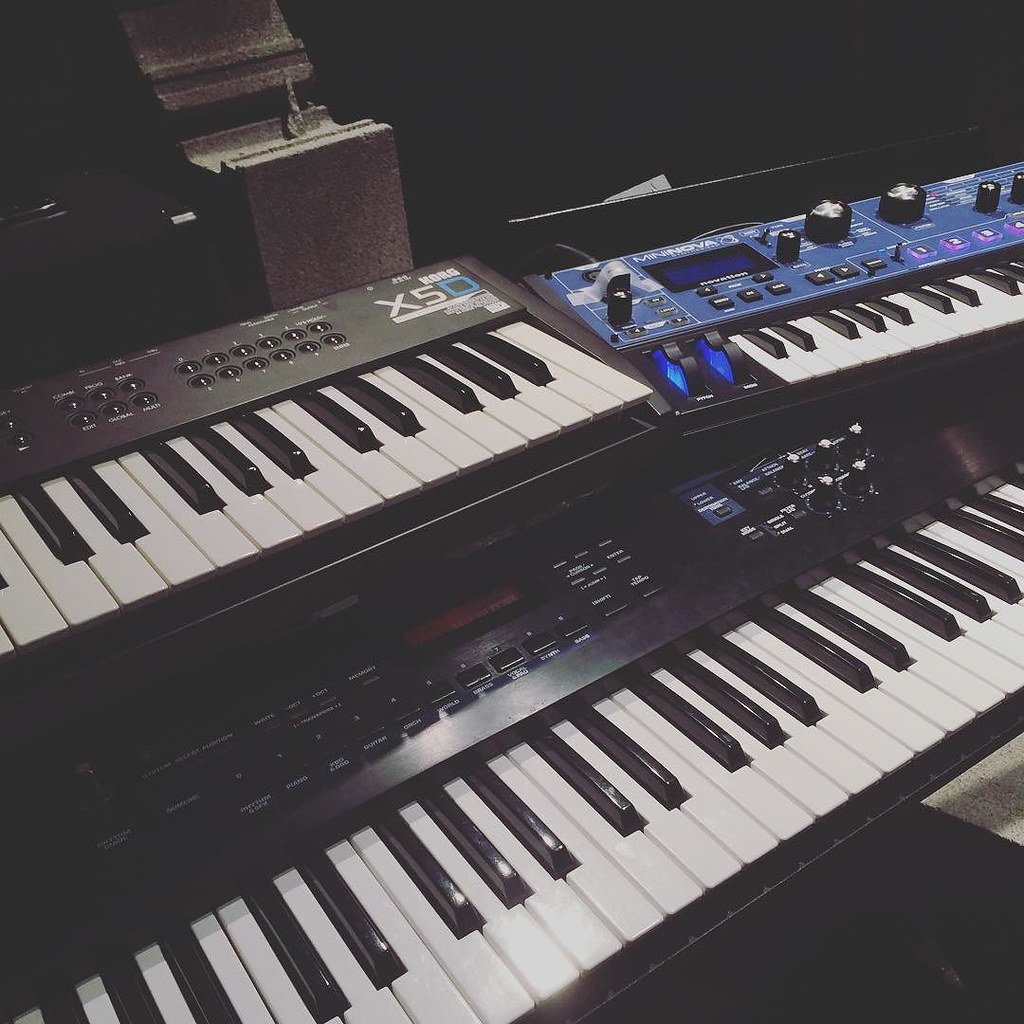This image features three professional-grade electric piano keyboards arranged in a stacked setup commonly seen at music concerts. The largest keyboard dominates the bottom of the frame and is a sleek black and white instrument with buttons rather than knobs. Positioned above it are two smaller keyboards. The one on the left, identifiable by the label "Korg X5D," sports a gray background and a mix of white and blue letters (X and 5 in white, 0 in blue). This keyboard is primarily black with white keys. On the right, there is a "Mininova" keyboard, which stands out with its blue background, abundant knobs, and a digital LED display on the far left. This instrument also features black and white keys but is more focused on sound mixing capabilities. All three keyboards present advanced features and are partially out of frame, suggesting a tight, immersive setup. The photo is taken at an angle, adding a dynamic perspective to the scene. There also appears to be a stool or piano bench underneath the larger keyboard at the bottom, adding to the concert-style arrangement.